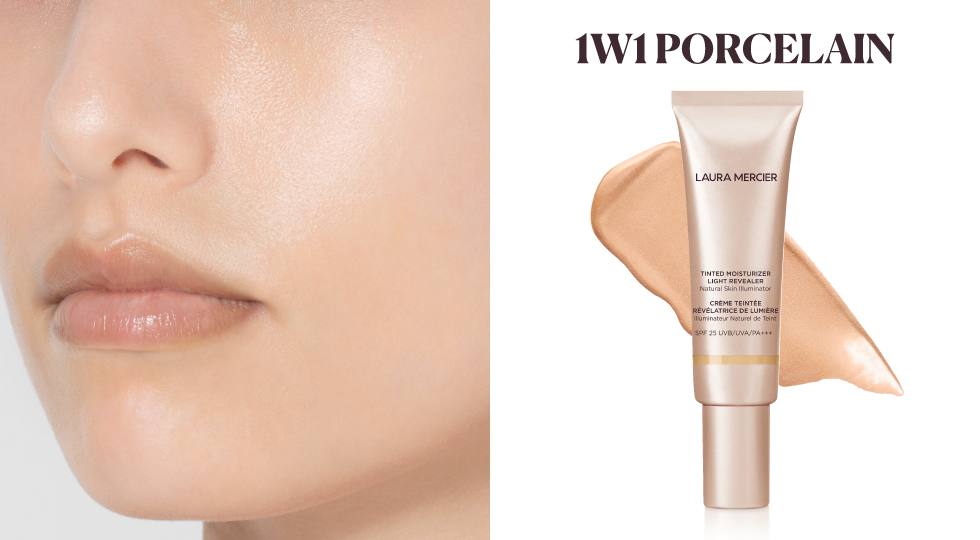This image is a detailed advertisement for Laura Mercier's Tinted Moisturizer Light Revealer Natural Skin Illuminator in the shade "1W1 Porcelain." The display is split into two sections. The left section prominently features a close-up photograph of a Caucasian woman's face, showcasing her flawless, radiant skin from just below the midpoint of her nose to slightly past her chin. She is angled to the side, highlighting her smooth cheek, the side of her nose, and her pink, glossy lips. The right section of the display highlights the product itself: a cream tube of the tinted moisturizer with the product name in both English and French. Behind the tube is a smear of the product, matching the woman's pale skin tone, with the shade name "1W1 Porcelain" displayed above in black text.